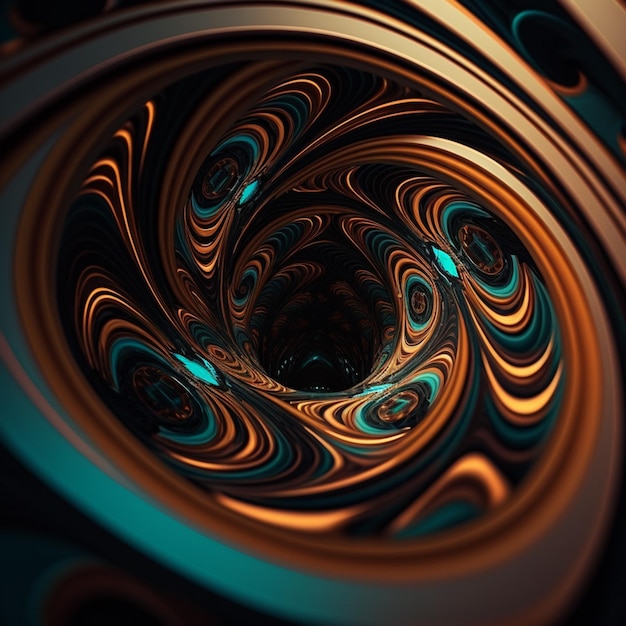The artwork is an abstract masterpiece, presented in a square format with sides of equal length. Dominated by a central, swirling tunnel, the image pulls the viewer into a mesmerizing vortex, featuring intricate designs that seem to blend and melt into one another. The tunnel is encircled by concentric layers of complex patterns: an inner black clock face with blue hour and minute hands, ensconced within a blue circle, followed by a series of three copper rings, and additional blue circles. The repetitive circles and patterns swirl and meld, creating an impression of a constantly moving, melting spiral. The outer regions of the tunnel showcase swirling ovals and bands in gold, teal, brown, and aquamarine colors, adding to the sense of motion and depth. These elements give way to a dark void at the center, evoking the feeling of staring into a never-ending spiral of time. A brass circle can be seen entering the tunnel at the top right, further adding to the intricacy and depth of the piece.